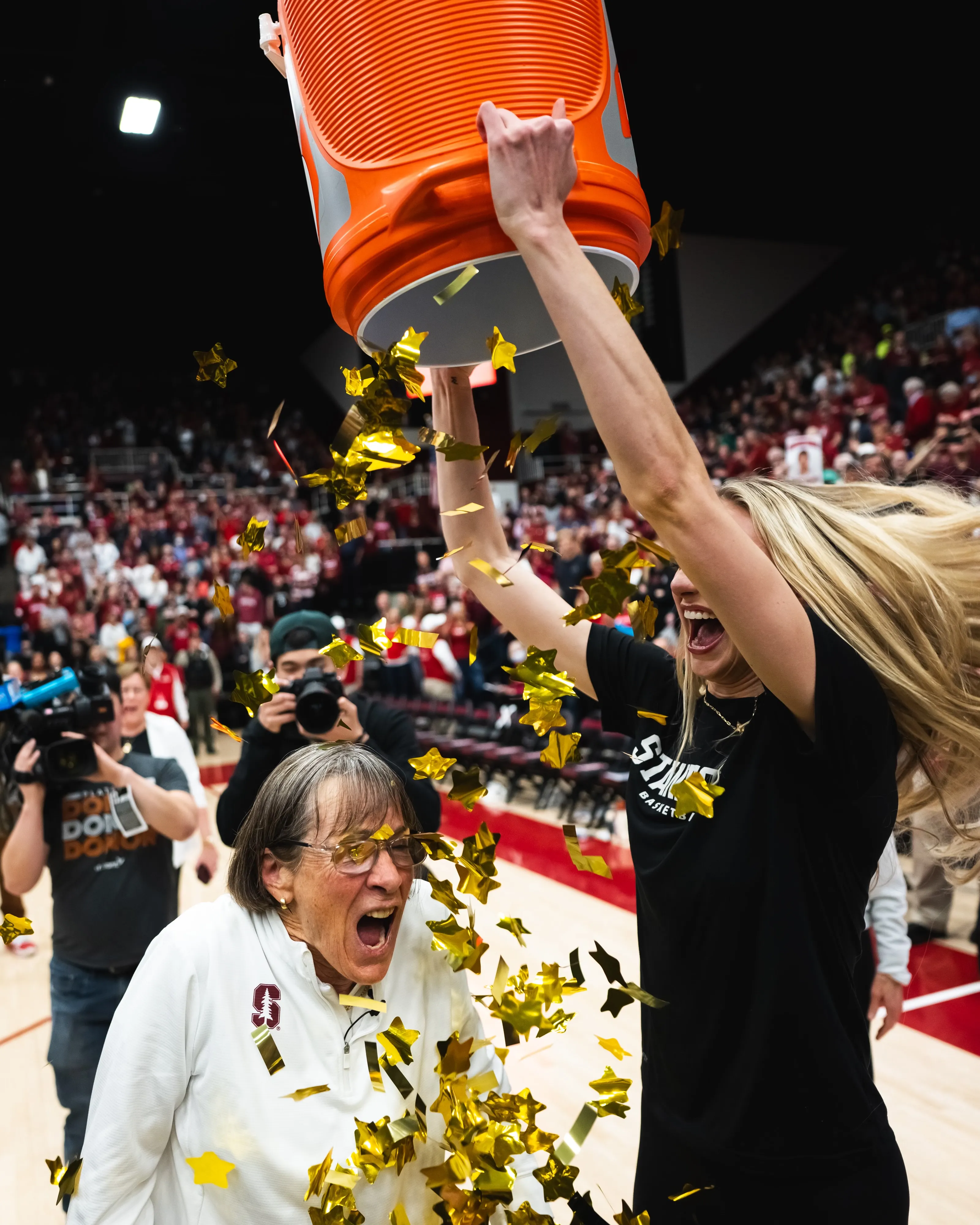The image captures a lively moment at a basketball game. The scene is set on the wooden court marked by a red-striped border, with a backdrop of a packed bleacher full of fans decked out in red t-shirts and waving white and red jerseys. Under the black ceiling spotlight, the central action unfolds between two women. A young blonde woman, wearing a black shirt emblazoned with the word "Stanford" in white, holds an orange Gatorade cooler upside down over the head of an older woman. Instead of liquid, the cooler releases a shower of golden star confetti. The older woman, donned in a white pullover sweater with a red "S" and a cedar tree emblem, stands with her mouth open in surprise and eyes widened behind glasses. Her short grayish-brown hair contrasts with her youthful, spirited reaction. Both women exude joy as photographers in the background, including a kid, capture the jubilant scene.